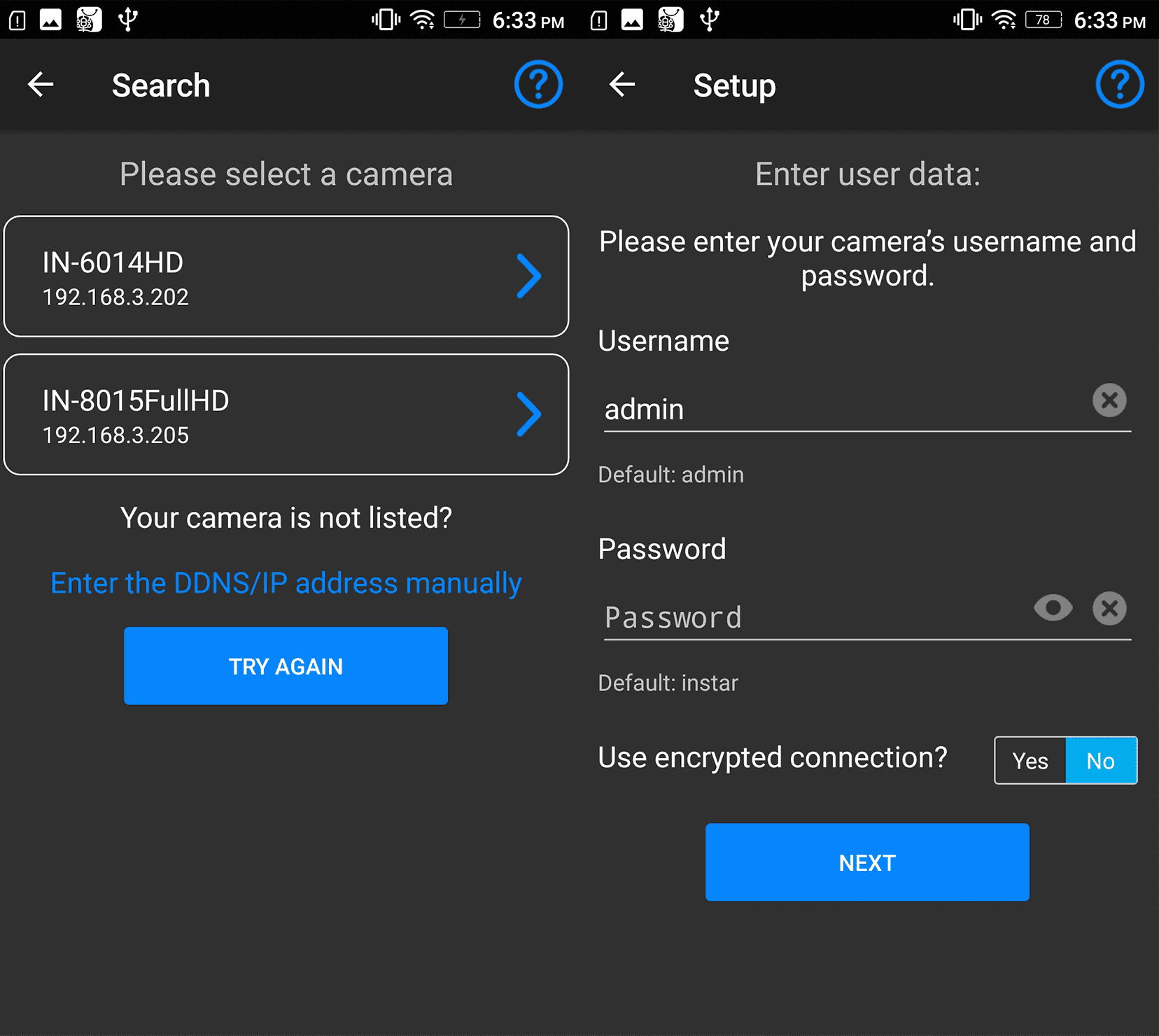This image shows two smartphone screens placed side by side, creating a composite view that resembles a large black square formed by two smaller rectangles. The screens display what appears to be a setup or configuration process for a digital camera system. The time on both screens is 6:33 p.m.

On the left screen, it shows a search interface with two options: "4 HD" and "Full HD," both presented under the prompt "Please select a camera." There is also a message that reads, "Your camera is not listed?" followed by "Enter the DDNS/IP address manually." A button labeled "Try Again" is found at the bottom of this screen. Additionally, a blue circle with a question mark icon is prominently featured.

The right screen is titled "Set Up" and prompts the user to "Enter user data." It has fields for "Username" and "Password." The default username is "admin," which can be edited or deleted using an adjacent X button. There is also an option to select "Use encrypted connection," with choices of "Yes" or "No." A "Next" button appears at the bottom of this screen. A matching blue question mark encased in a blue circle is also present on this screen, indicating potential help or information is available.